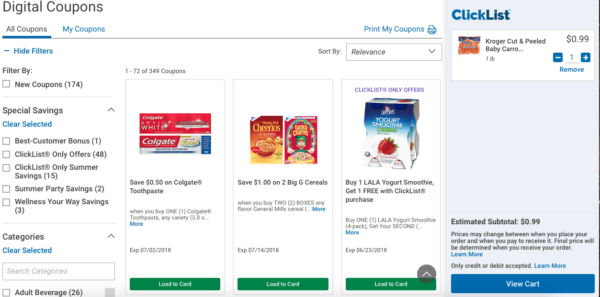The webpage displays digital coupons available to a specific user. The layout is divided into two main sections:

### Left Section (Two-thirds of the Page)
- **Title:** "Digital Coupons"
- **Tabs:** 
  - "All Coupons" (currently selected)
  - "My Coupons"
- **Filter Bar:** Located on the left side with options to filter by:
  - New Coupons
  - Special Savings (with quantities in parentheses):
    - Best Customer Bonus
    - Checklist Only Offers (48)
    - Clicklist Only Summer Savings (15)
    - Summer Party Savings (2)
    - Wellness Your Way Savings (3)
- **Category Search Bar:** At the bottom left for searching by categories
- **Displayed Coupons:** Three coupons listed with the following details:
  - **Product Name:** Colgate
  - **Product Name:** Big G Cereals
  - **Product Name:** Lala Yogurt Smoothie
  - Each includes an image, the savings amount, disclaimer text, expiration dates, and a green "Load To Carts" action button

### Right Section (One-third of the Page)
- **Light Blue Background Box** with a colorful "Quick Click List" logo in the upper left
- **Displayed Item:**
  - **Product:** Kroger Cut and Peeled Baby Carrots (1 pound)
  - **Image:** Small picture of a bag of carrots
  - **Price:** $0.99
  - **Quantity Adjustment:** 
    - Minus arrow in a blue square
    - Plus arrow in a blue square
    - Centered quantity number ("1")
    - "Remove" button underneath
  - **Estimated Subtotal:** $0.99
  - **Disclaimer Text:** "Prices may change between when you place your order and when you pay to receive it. The final price will be determined when you receive your order."
  - **Links:** "Learn More" (in blue) and "Only Credits or Debits Accepted"
  - **Action Button:** "View Cart" at the bottom

The webpage is designed to facilitate easy navigation and selection of digital coupons, with the option to view detailed information and adjust quantities for specific items.